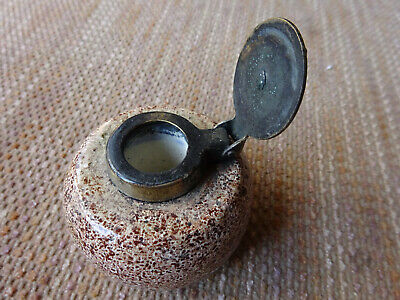The photograph showcases a small, cylindrical container resting on a textured, multi-toned surface. The surface, which could be a bumpy table, braided placemat, or stone-like macrame, features a palette of white, light brown, dark brown, and hints of cream, blue, and lilac, contributing to a natural aesthetic. The container itself is similarly hued in white and light brown, closely blending with the background. It is a small, rounded jar, capable of holding approximately one-third of a cup of liquid. The jar is topped with a dark, possibly rusted metal or black lid featuring a circular handle and a clasp mechanism that is currently open, hinting at its use for securely enclosing the container’s contents. The intricate details of both the surface and jar create a harmonious, earthy visual composition.